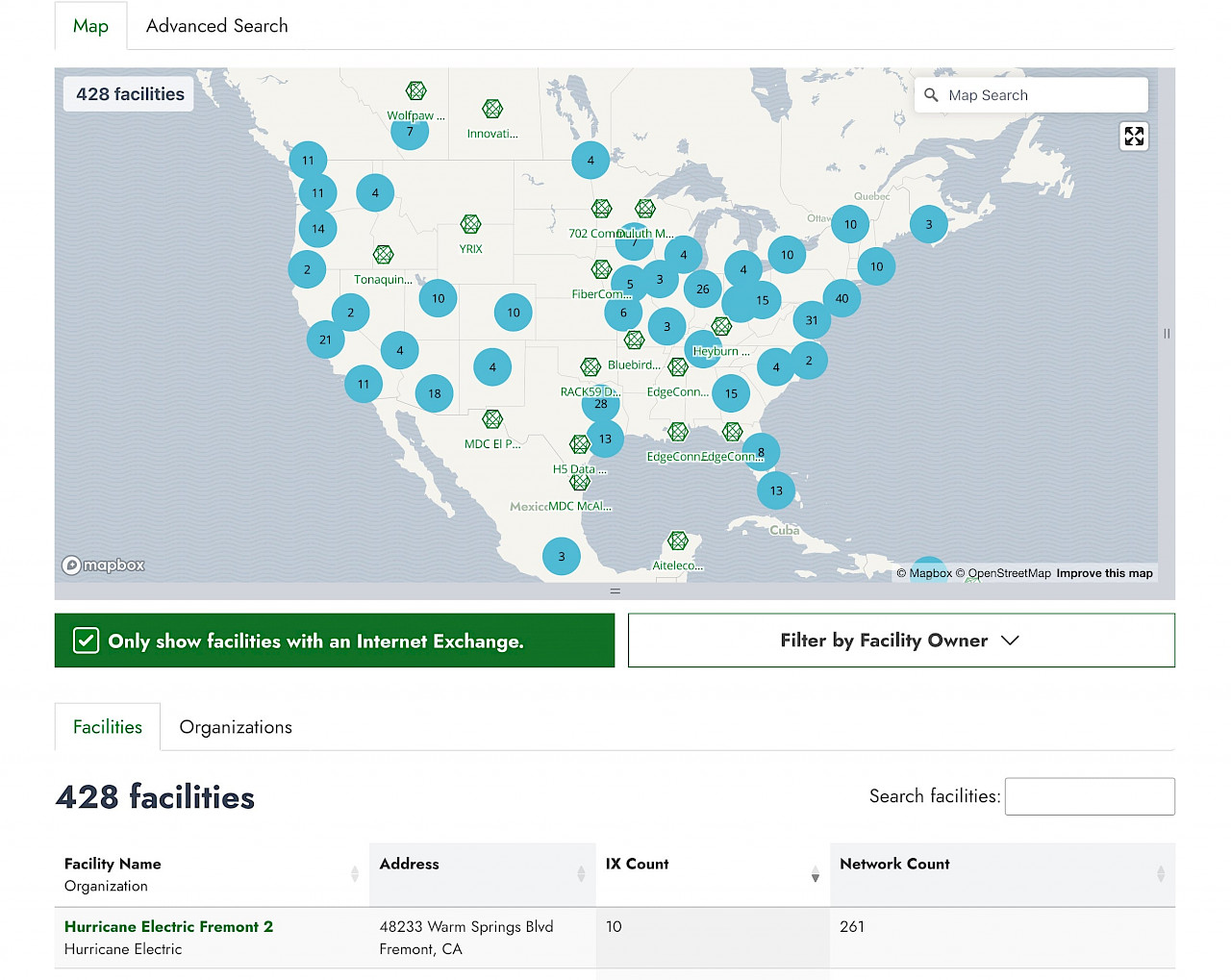In the image, we see a detailed, computer-generated map of the United States, which is depicted in a light gray color against a regular gray background. The map is dotted with blue circles, each containing a number, representing specific data points across various regions. In the top-left corner of the image, text indicates "428 facilities," while the top-right corner features a search bar labeled "map search."

Below the map, in a green rectangular box, there is an option that reads "Only show facilities with an internet exchange." Adjacent to this, on the right-hand side, black text instructs "filter by facility owner."

At the bottom of the image, there are two tabs: the left tab labeled "facilities" and the right tab labeled "organizations." The sections within the bottom area include columns titled "facility name," "address," "IX count," and "network count," each filled with corresponding information. The background colors under these details vary, with a couple of sections displaying a gray background, two sections with a white background, and three sections with a light gray background.

Additionally, there is another search bar option labeled "search facilities" located above the detailed sections on the right side of the image, completing the comprehensive visual data representation.